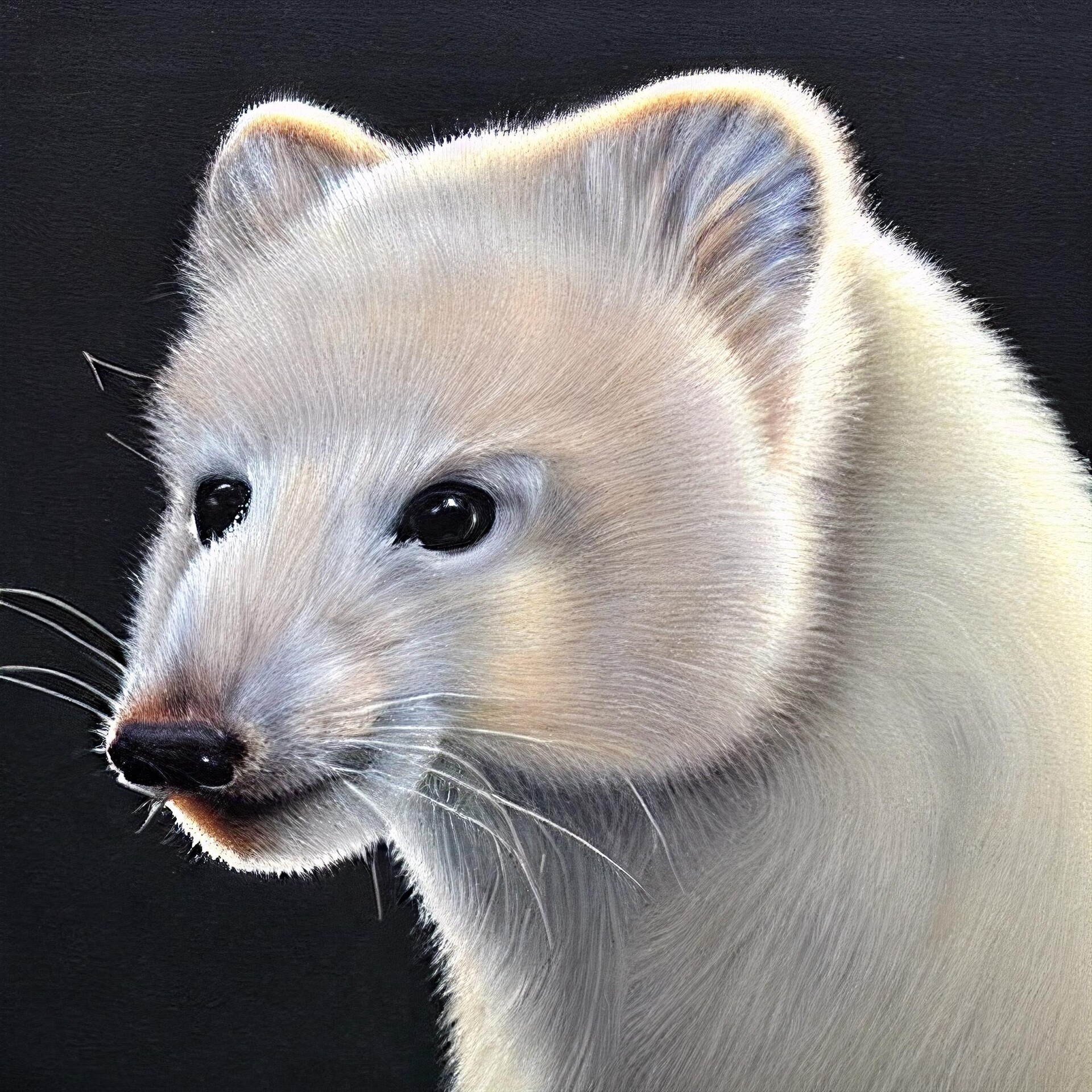The image is a detailed, realistic painting of a white weasel, set against a solid black background. The creature, facing slightly to the left, is depicted from the head down to the upper part of the body, ending around the chest area. It has rounded triangular ears and big, black, beady eyes. The weasel’s pointed snout is adorned with a black nose, and white whiskers extend from its muzzle. Small round ears and a dense coat of white fur cover its entire body, with slight brownish patches around the nose and sometimes the mouth, accentuating its features. The individual white hairs and fur directions are meticulously painted, showing how they swirl upwards and to the sides. Shadows beneath its chin and neck add depth, while the stark black background makes the detailed fur and whiskers stand out brilliantly. Overall, the weasel's expression is neutral, almost serene, giving it an adorable but solid look.